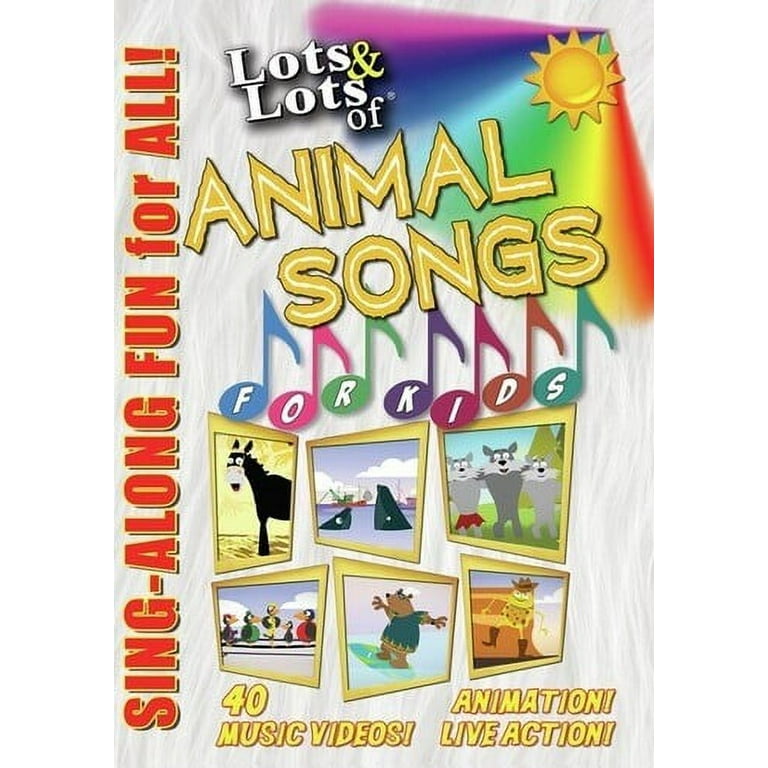The image is a vertically aligned rectangular cover for a sing-along video for kids. Along the left-hand side, the text "Sing-along fun for all!" is written in large, reddish-orange letters outlined in gold, starting from the bottom and going up. The background features a curvy pattern of white and gray. 

At the top center, the text "Lots and lots of animal songs" is prominently displayed, with "lots and lots of" in white and "animal songs" in yellow with a lighter yellow center. In the top right corner, an image of a sun with a rainbow canopy spreading from it symbolizes happiness and joy.

Across the center, musical notes appear in various colors including blue, pink, green, purple, violet, brown, and green. The circular parts of these musical notes contain the words "for kids" in white letters. Below these notes are six images of different cartoon animals such as a horse, some rams, wolves, birds on a line, and a bear surfing.

Finally, towards the bottom of the image, the text "40 music videos, animation, live action!" is written in yellow. This comprehensive cover combines vibrant visuals and engaging text to attract children to an entertaining sing-along experience filled with animal-themed fun and music.